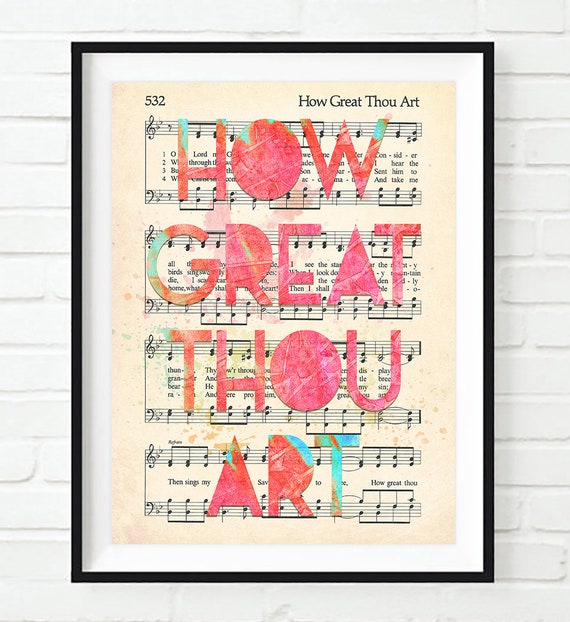The photograph features a vintage-looking sheet music of "How Great Thou Art," framed in a thin black border. The sheet, marked with "532" on the top left, is an off-white or cream color, giving it an antique appearance. Black musical notes span the entire page, and the title, "How Great Thou Art," is prominently displayed at the top right. Overlaid on top of the music notes, there is an artistic touch with the words "How Great Thou Art" seemingly painted in a striking pink hue, accented with green on some letters, and a hint of blue on the last letter. The sheet music rests against a plain white background and the entire piece is mounted against a painted white brick wall. This carefully crafted artwork merges the traditional with the modern, creating a harmonious and visually captivating tribute to the timeless hymn.